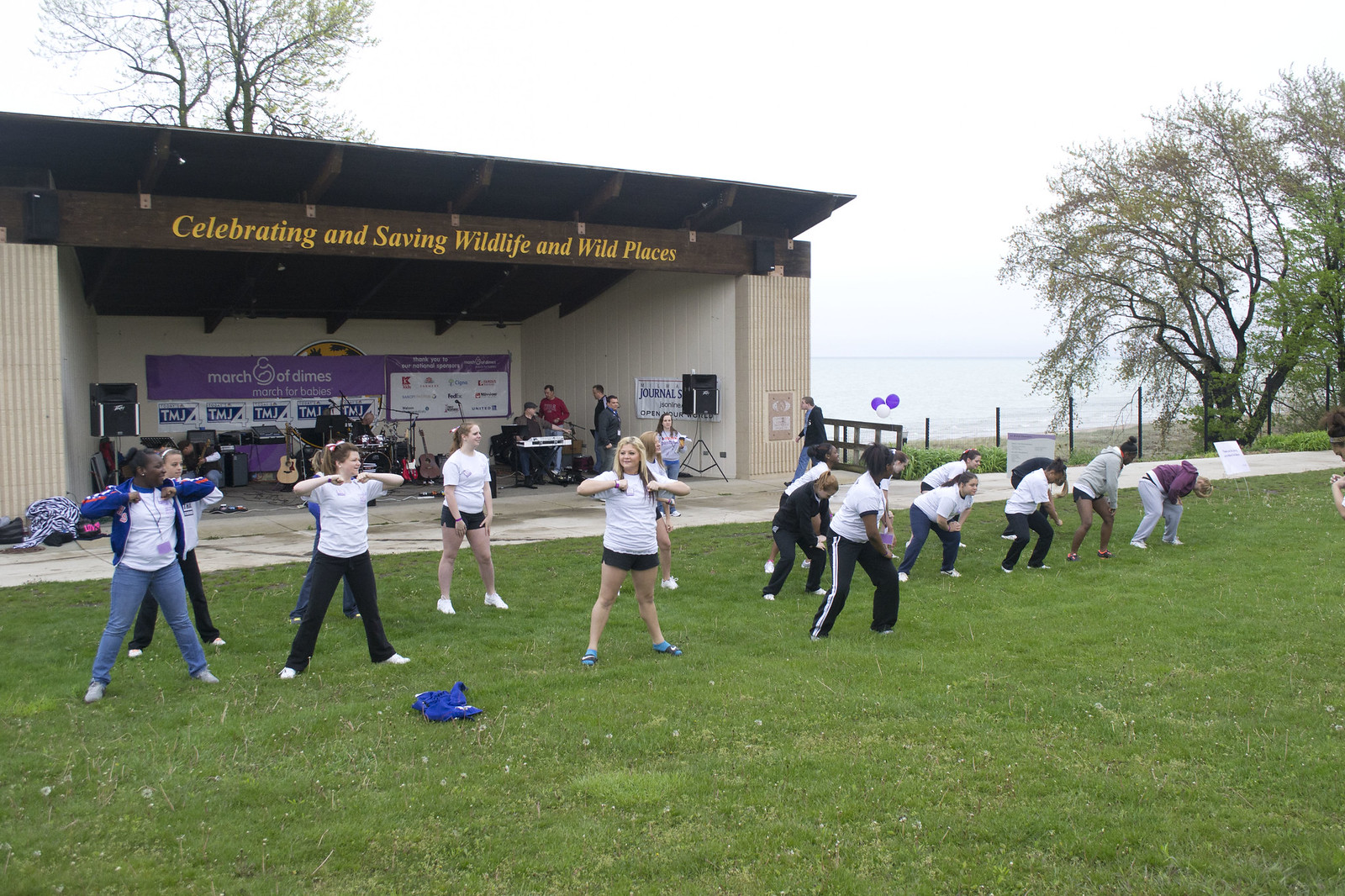This color photograph captures a lively outdoor scene beside a beach or lake, showcasing a group of individuals, predominantly women, engaging in a mix of dance routines and aerobic exercises on a grassy field. Each person is adorned in a white t-shirt paired with either black pants, shorts, jeans, or jackets, indicating a cool, overcast day with diverse weather-appropriate attire. The dancers are positioned in various dynamic postures, suggesting either a cohesive performance or individual routines.

In the background stands a bandshell with a slanted roof supported by vertical columns, framed by a large tree to the right. The band's presence is highlighted by visible instruments like a drum set and guitars, with banners inside the bandshell promoting 'March of Dimes, March for Babies, TMJ.' Over the stage opening is a prominent banner declaring, 'Celebrating and saving wildlife and wild places.'

Scattered around are bags and vibrant purple and white balloons, adding to the festive atmosphere. A road separates the grassy performance area from the bandshell, where a diverse crowd, including passersby, enhances the communal vibe of this vibrant event.